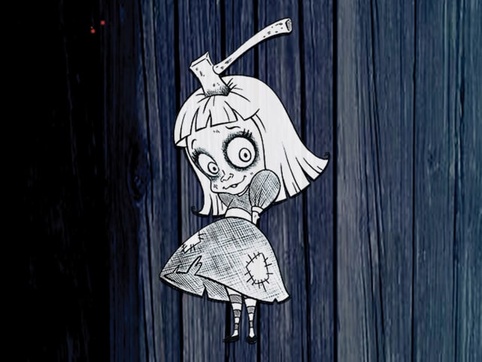The image showcases a striking black and white graffiti artwork, possibly done with pen and ink, that is pasted on weathered wooden planks, appearing in shades of black, dark gray, and brown. The focal point is a cartoon depiction of a young girl, reminiscent of Tim Burton’s style, with large, expressive eyes and shoulder-length blonde hair with short bangs. She wears a raggedy dress adorned with patches and has striped tights paired with small black dress shoes or ballet flats. Despite the unsettling hatchet embedded in the top of her skull, her expression remains surprisingly calm and unbothered, adding a curious juxtaposition to the scene. The overall effect is haunting yet endearing, inviting viewers to ponder the deeper meaning behind the imagery.